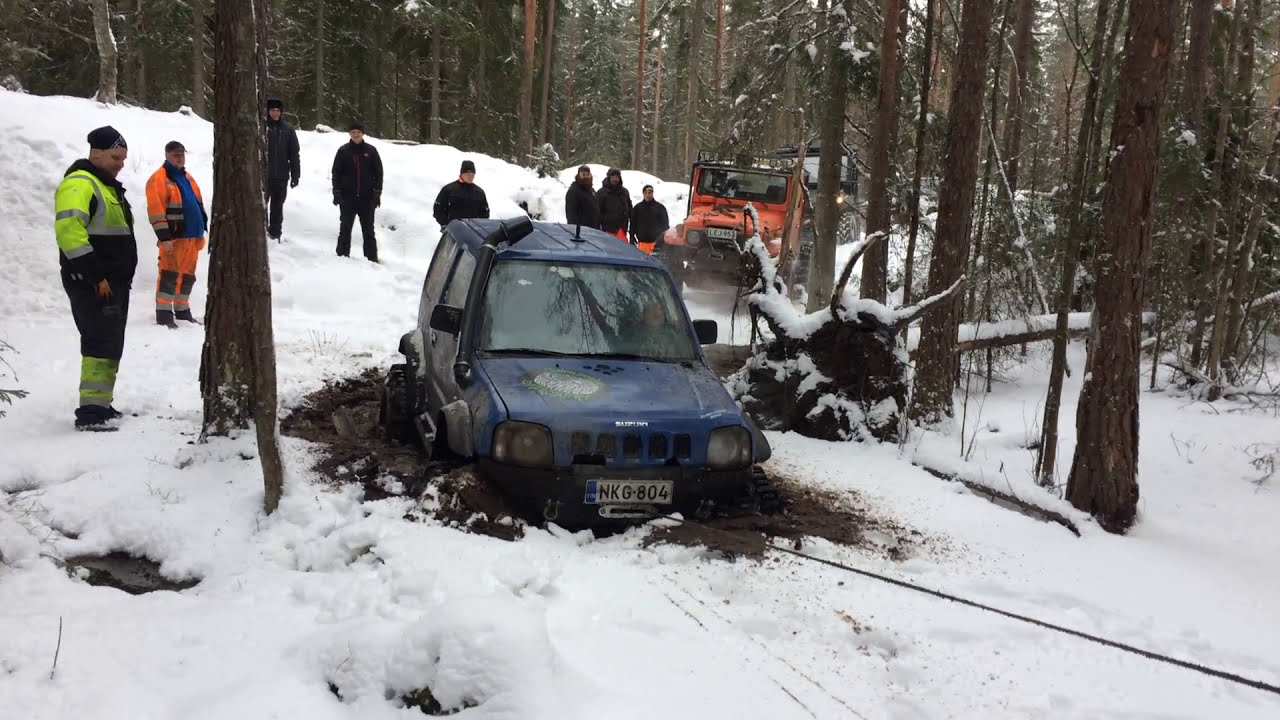In this photograph, we see a vehicle rescue operation underway in a snowy, wooded area during daylight. At the center of the image is a blue SUV, half-submerged in muddy water, indicating it may have been stuck for some time. The vehicle has a license plate reading NKG-804. A rope or line is attached to the front, suggesting efforts to pull it out. Surrounding the SUV are several men, presumably rescue workers, closely monitoring the situation. On the left side of the image, a man in a safety yellow jacket with reflective yellow on the upper part and calves, and black in the midsection, can be seen. Just to the right of him stands another man in similar reflective gear, but in neon orange. Further in the background, partially obscured by the scene's primary focus, is an orange Jeep. The landscape features a dirt hill covered in snow, leading into a dense forest with various hues of brown and green. The collective colors within the image include white, the neon hues of rescue gear, and the natural tones of the environment, painting a vivid scene of this wintry vehicle recovery mission.